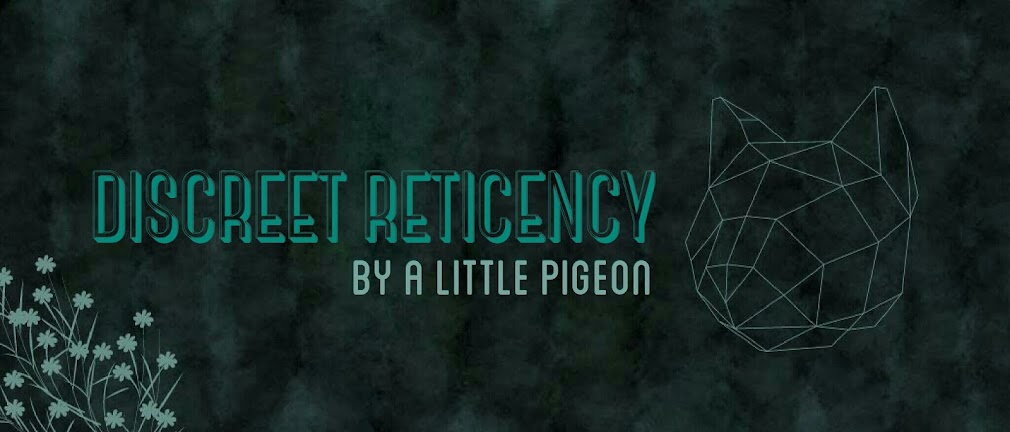The image features a dark, mottled background comprised of black, gray, green, and blue streaks. In the bottom left corner, there are light green and blue flowers with an abstract design, consisting of circular shapes with small ovals branching out from them, resembling daisies but without leaves. Positioned in the center left of the image is the title "Discreet Reticency," spelled R-E-T-I-C-E-N-C-Y in three-dimensional blue and black text. Directly beneath this title is the phrase "by a little pigeon," written in white text. On the right side of the image, there is a digital, vector-style line drawing depicting the head of a cat or tiger, composed of interconnected geometric shapes such as squares, rectangles, and triangles. The overall composition gives a striking blend of abstract and digital art elements against a textured, mixed-color backdrop.